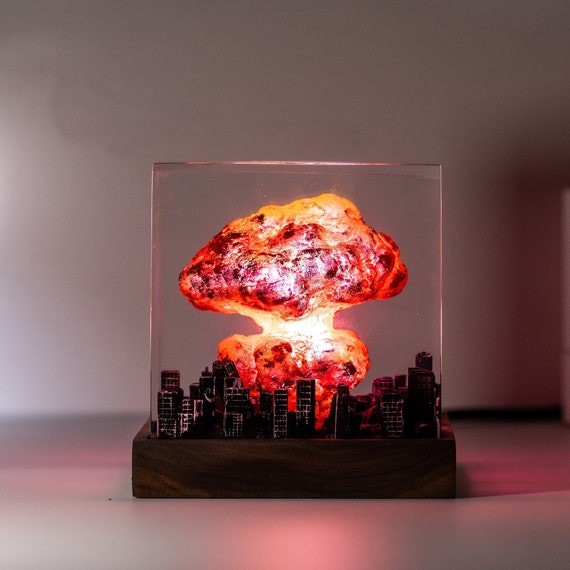The image is a photograph of an art piece designed as a model or diorama. This detailed work of art is set on a smooth beige surface with a white background. Encased in a clear, vertical square glass case, the model features a city skyline reminiscent of New York, with black skyscrapers accented by gold to simulate illuminated windows. Central to this urban scene is a dramatic depiction of a nuclear explosion, showcasing a towering mushroom cloud. The explosion is a striking combination of colors: a smaller red mushroom cloud rises initially, followed by a larger one above it, transitioning from bright yellow at the core to red and orange hues, with flecks of bright white and gold highlighting the impact. This intricate display, framed at the base by a dark brown wooden border, creates a captivating and chilling representation of a city under nuclear attack.